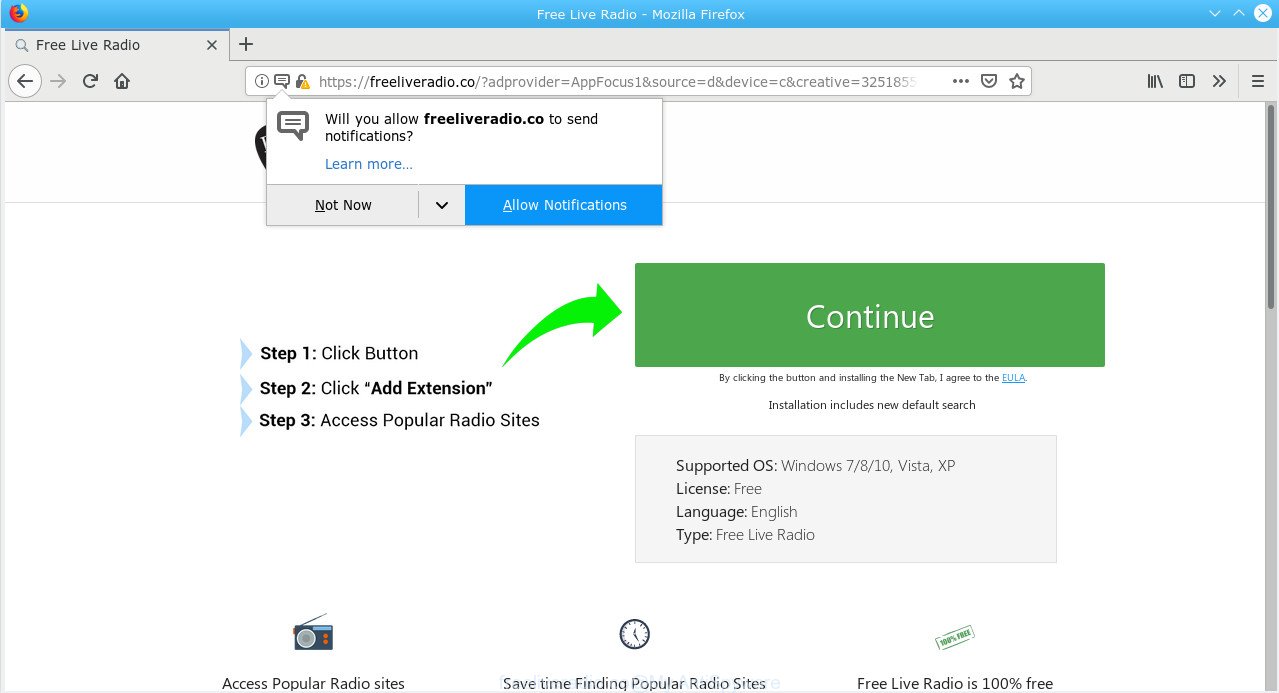The screenshot displays an older version of Mozilla Firefox with a simplistic, somewhat dated interface. At the top, there is a light blue navigation bar, contrasting with the otherwise grey browser frame. The main content area of the browser shows a white webpage from "freeliveradio.co," as indicated by the address bar. However, the title and logo of the page are partially obscured by a Firefox notification asking whether to allow freeliveradio.co to send notifications, with options to either click "Not Now" or "Allow."

The visible portion of the webpage appears to be a download or installation guide, prominently featuring a series of steps. Step 1 instructs users to click a button, Step 2 to click "Add extension," and Step 3 promises access to popular radio sites. A large green arrow directs attention to a conspicuous "Continue" button on the right. Beneath this button, a disclaimer clarifies that by clicking it and installing the new tab, the user agrees to the End User License Agreement (EULA). Additional information at the bottom of the page outlines system requirements and supported operating systems, listing Windows 7, 8, and 10, with the service being described as free and available in English.